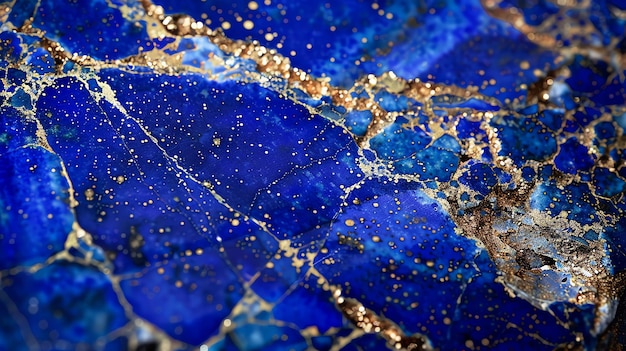The photograph captures a close-up, highly detailed image of a striking blue surface, likely a precious stone such as lapis lazuli or a piece of ceramic pottery. The dominant hues range from dark indigo to lighter, almost white blues, creating a vivid background. Interwoven throughout the blue are intricate, golden veins and speckles that vary in thickness and density. These veins give the appearance of melted gold that has filled in the cracks of the stone or pottery, adding a sense of value and beauty to the image. The golden material also forms delicate lines and dots, sometimes concentrating more heavily in certain areas and shimmering like fine gold dust. The image is slightly blurred at the top right and bottom left corners, enhancing the abstract, almost mosaic-like quality of the composition. Overall, the interplay between the blue and gold, along with the presence of browns and beiges in the cracks, renders a mesmerizing and valuable visual experience reminiscent of a stained glass mirror.